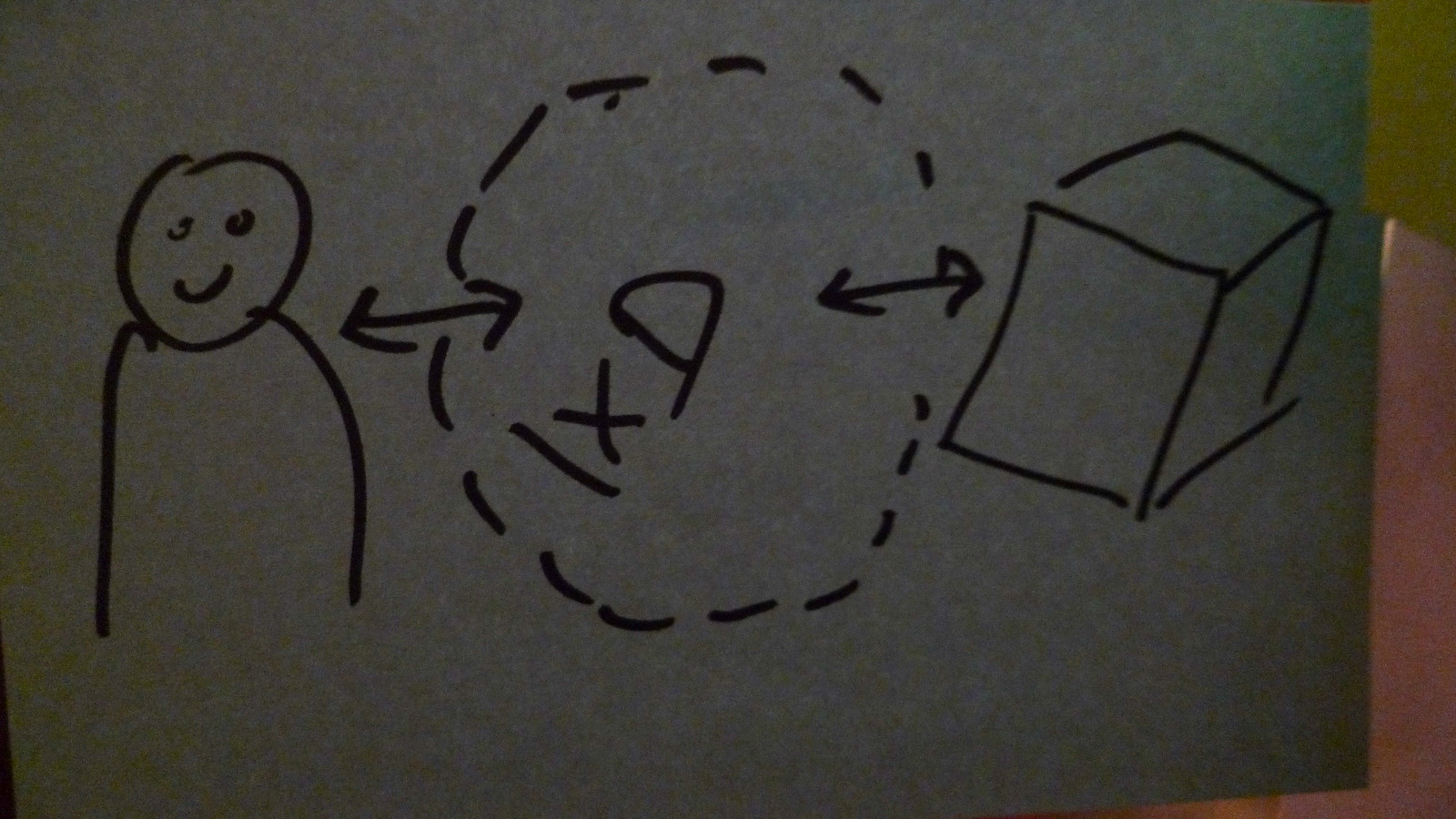A hand holds a white piece of paper featuring a drawing created with a black marker. The drawing depicts a smiling person with two eyes and no ears or arms. Positioned to the right are two arrows, pointed horizontally from left to right, and in between them lies an angular, dotted circle. On the far right side of the paper, there is a 3D, right-tilted square box. The notation "1 x d" is written below the person, also tilted, accompanying the horizontal arrows and the angular circle. The background reveals a yellow wall, suggesting an indoor setting. The image appears grainy, indicating that it was taken in low light conditions. The overall composition on the paper is casual and imperfect, conveying a sense of informal, hand-drawn creativity.